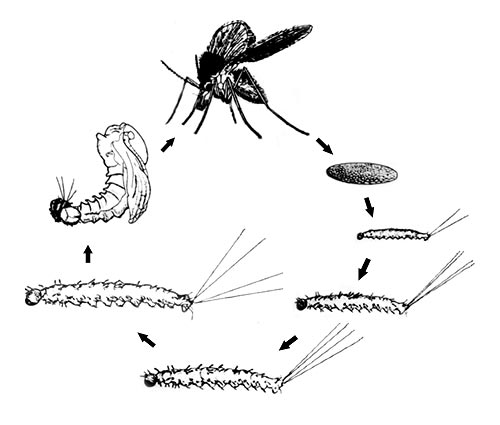This image is an intricate black and white diagram illustrating the life cycle of a mosquito against a plain white background. The diagram is arranged in a circular, clockwise flow with arrows connecting six distinct phases. At the top is the full-sized adult mosquito. Moving to the right, the first phase is a small, oval-shaped egg laid by the mosquito. It then shows the hatching of the egg into a small larva, depicted with two antennae. The stages progress with the larva growing larger and acquiring four antennae, becoming more elongated. Subsequently, the larva transitions into a pupa, where wings start to emerge from its shell. The final stage completes the cycle, returning to the adult mosquito at the top. The detailed representation captures the entire developmental journey from egg to mature mosquito.